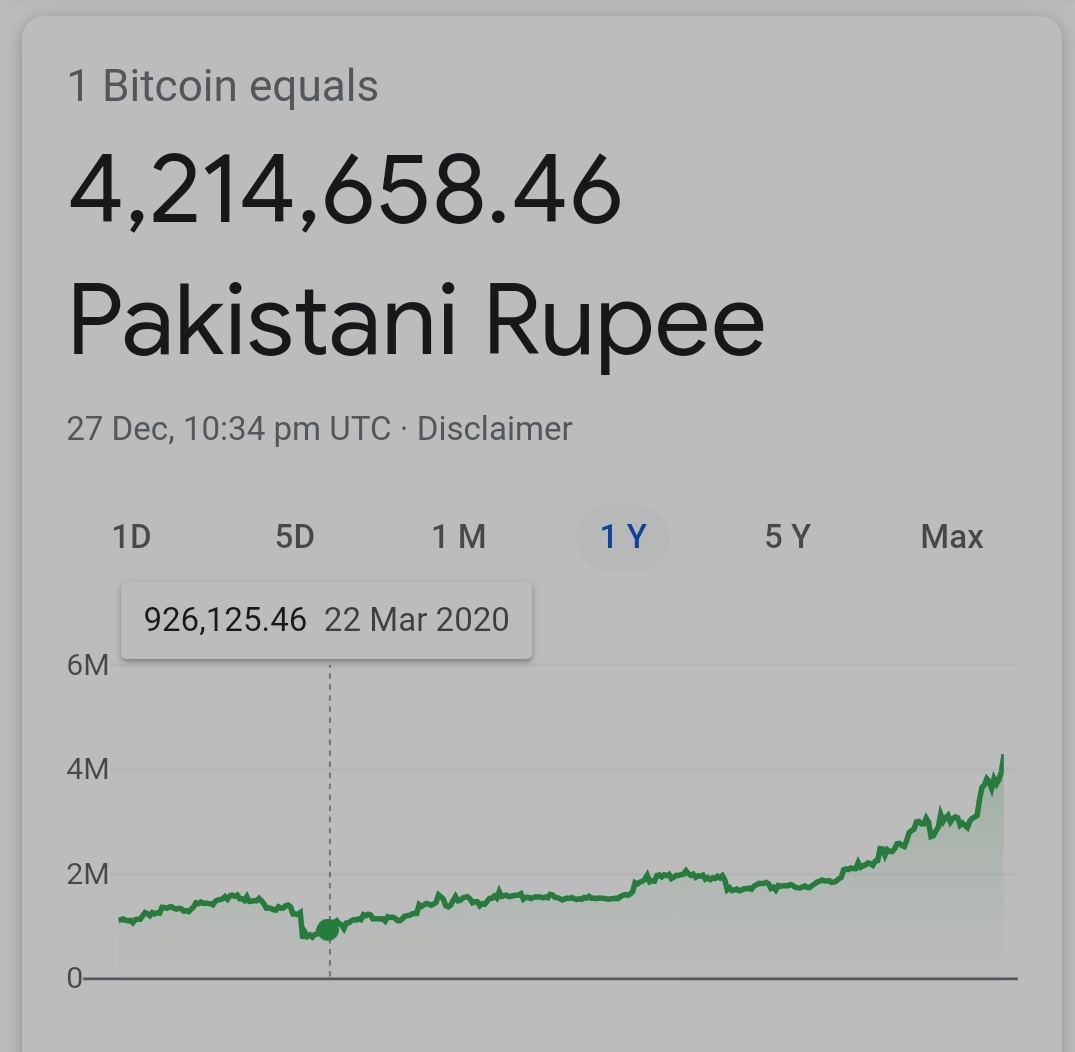A detailed and cleanly formulated descriptive caption for the image:

---

The image is a screenshot of a Google search result displaying the conversion rate of Bitcoin to Pakistani Rupee. At the top, there is a line of grey text indicating "1 Bitcoin equals." Below this, in much larger black text, is the conversion result: "4,214,658.46," followed by "Pakistani Rupee". This indicates that one Bitcoin is equivalent to 4,214,658.46 Pakistani Rupees. Underneath, a small line of text reads "27th of December, 10:34 PM UTC, disclaimer," showing the specific date and time when the conversion rate was accurate.

The bottom half of the image features a graph that tracks the conversion rate over different time periods, with "1 day," "5 day," "1 month," "1 year," "5 year," and "max" labeled on the x-axis. The "1 year" period is highlighted in blue, indicating that the graph displays the conversion rate over the past year. On the y-axis, the values are marked at intervals of zero, two million, four million, and six million, illustrating the price trend of Bitcoin relative to the Pakistani Rupee. The graph curves upward, suggesting an increase in Bitcoin's value over the year. One data point on the graph is specifically highlighted in yellow, showing a value of "926,125.46" on the 22nd of March, 2020, indicating a significant point in the yearly trend. The line of the graph itself is shown in green, marking the gradual rise in Bitcoin's value throughout the year.